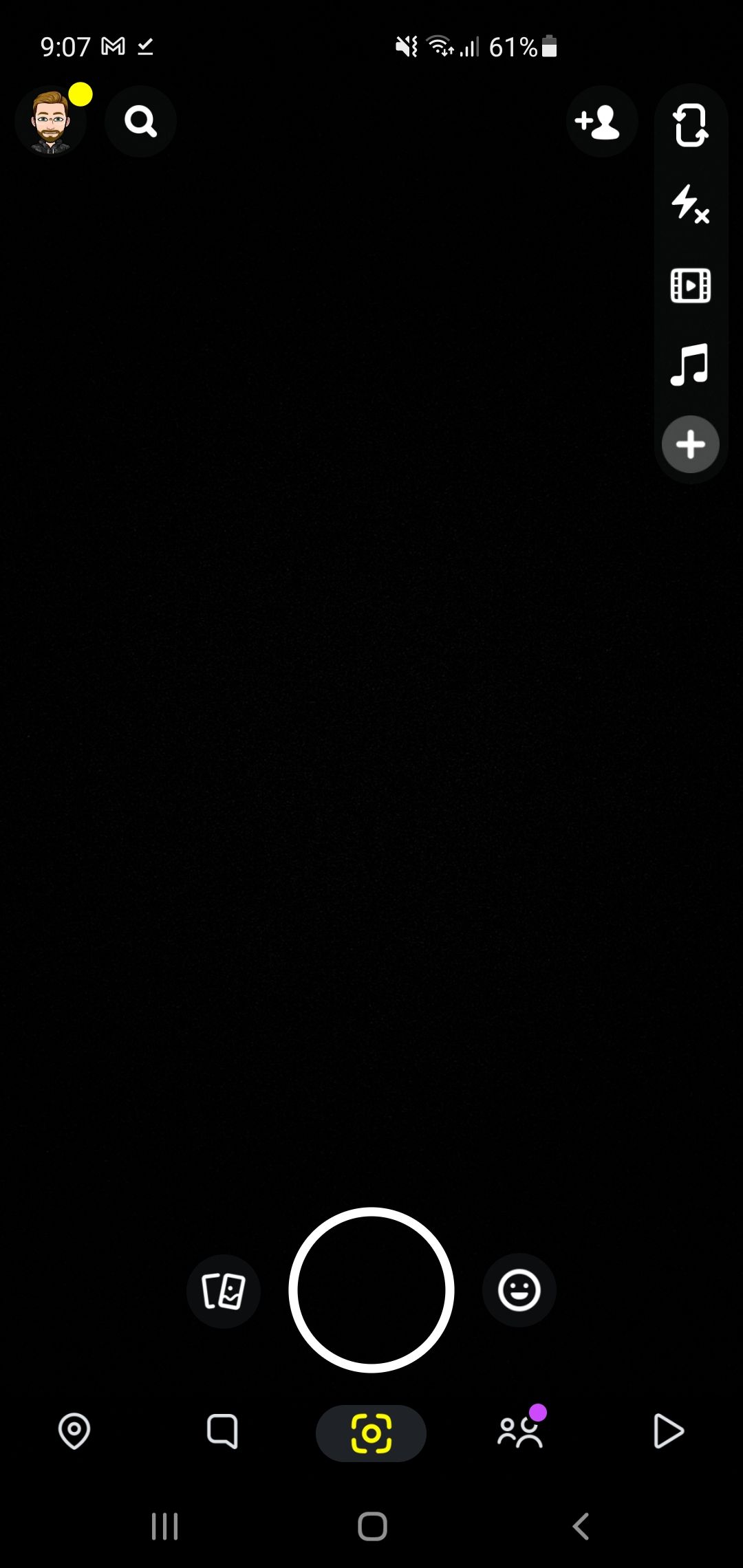This image depicts a screenshot of an Android mobile device displaying the Snapchat app interface. At the top of the screen, the status bar features various notification icons, including one for Gmail, a mute icon, Wi-Fi signal strength indicator, network signal bars, and the battery indicator showing a 61% charge remaining. Below the status bar, the Snapchat app's interface includes the rotate camera icon, an add music button, and the large, circular camera shutter button. The rest of the screen behind these icons is black and blank, indicating that the camera is not actively capturing any visual content at the moment.